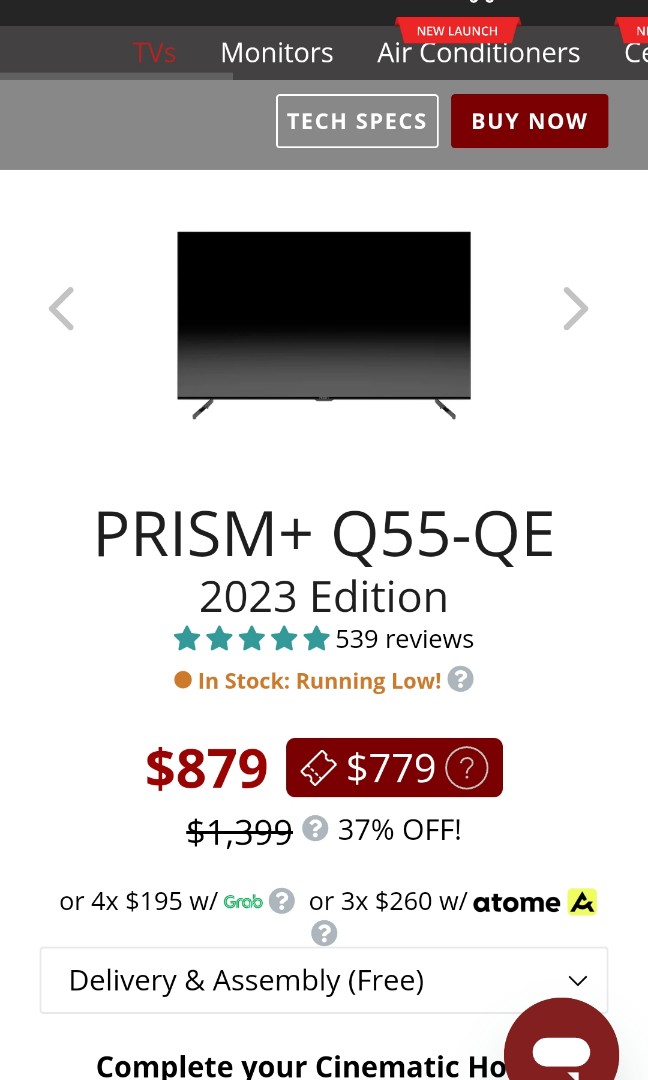This is a detailed screenshot of an advertisement for the Prism Q55-QE flat screen television, the 2023 edition. The top section of the screenshot features a black border with browse categories, including TVs, monitors, and air conditioners. The highlighted item, the Prism Q55-QE, boasts 539 customer reviews. The TV is currently on sale for $879, prominently displayed as the primary price. However, within a red rectangular box featuring a ticket stub icon, a discounted price of $779 is listed, indicating a special offer for club members. This suggests that customers with a club membership can purchase the TV at the reduced price of $779.